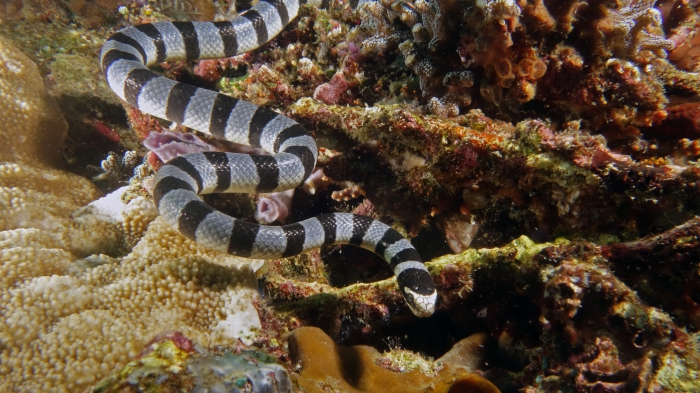The image showcases a gray and black striped snake, which appears to be underwater, slithering through a vibrant coral reef. The snake starts from the top left of the image, zigzagging three times in a wavy pattern—left, right, left, right—before its head points downwards near the bottom center of the frame. The snake's head is white at the tip, with a black band around its eyes, and one visible black eyeball. The snake’s scales are visible within the gray sections, which are slightly larger compared to the black bands.

The coral reef habitat beneath the snake features a diverse and colorful array of corals and marine life. On the left, there is yellow coral with white dots. The center displays a multicolored patch of reds, oranges, browns, greens, and yellows, while the right side includes larger, browner coral chunks. The overall scene is rich in color, ranging from green and yellow to purple, and other vibrant hues, suggesting a healthy and thriving underwater ecosystem. Despite the vivid description, the image's lighting and appearance hint that it may be either an image from a textbook or a photoshopped composition.